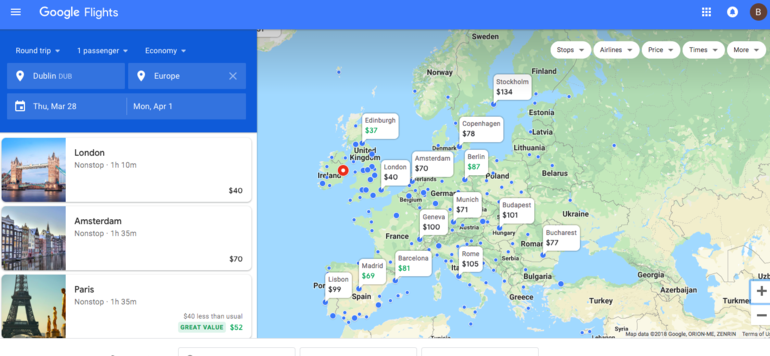The image shows the Google Flights website interface on which flight search results are displayed. On the left side of the screen, there are options for a round trip with one passenger indicated, alongside a tag labeled "ACOTV." There are two text fields visible: the first one at the top shows the departure location as Dublin on the left, and the destination as Europe on the right. The travel dates are set for March 28th to April 1st. Below this, three flight options are presented:

1. London: A non-stop flight with a duration of 1 hour and 10 minutes, priced at $40.
2. Amsterdam: A non-stop flight lasting 1 hour and 35 minutes, costing $70.
3. Paris: Another non-stop flight with a duration indicated as 1 hour and 35 am.

On the right side of the screen, there is a map of Europe marked with various location pins.